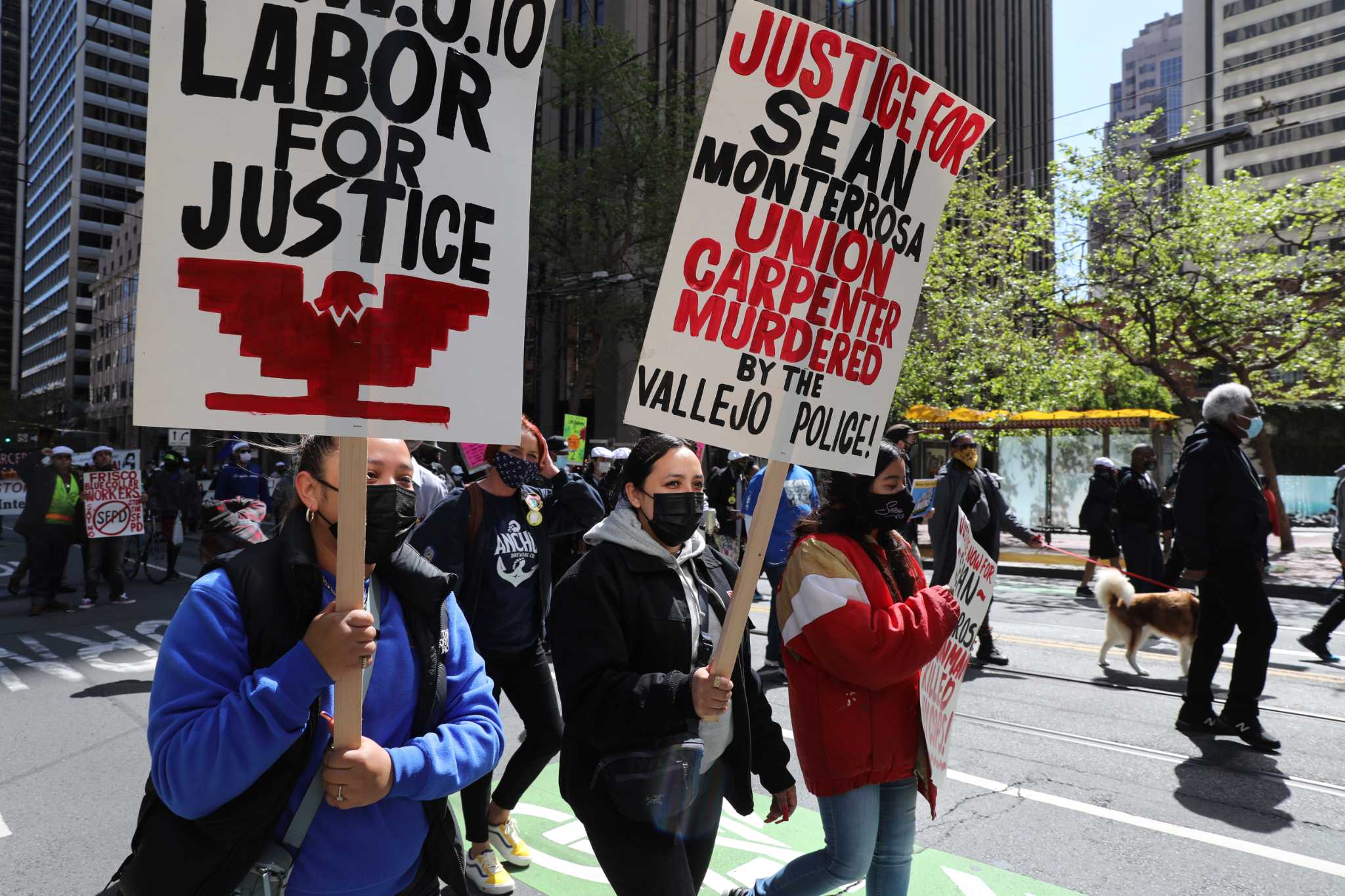The image depicts a peaceful protest march taking place on the streets of San Francisco during the COVID era, evidenced by the participants wearing facial masks. The focal point of the image is three young women marching in the middle of an asphalt street, surrounded by other protesters. The women are dressed in warm clothing, suggesting a fall or winter setting. They are each holding large white handmade signs. The woman on the left is wearing a blue long-sleeve shirt and a black vest and holds a sign with a red Native-looking eagle emblem that reads "Labor for Justice." The woman in the middle, dressed in a gray hoodie with a black jacket, carries a sign stating "Justice for Shawn Monterrosa, Union Carpenter Murdered by the Vallejo Police." The third woman, wearing a red, gold, and white jacket, holds a sign with red and black lettering that is partially obscured. The background reveals tall skyscrapers, a bus stop, and possibly a city park, indicating a large urban environment. Other protesters, some with their dogs, are visible carrying various signs, including one that says "Frisco Blue Collar Workers" with a crossed-out "SFPD" logo. The street features green imagery for bike lanes with clear white lines and text, underscoring the city setting of the protest.